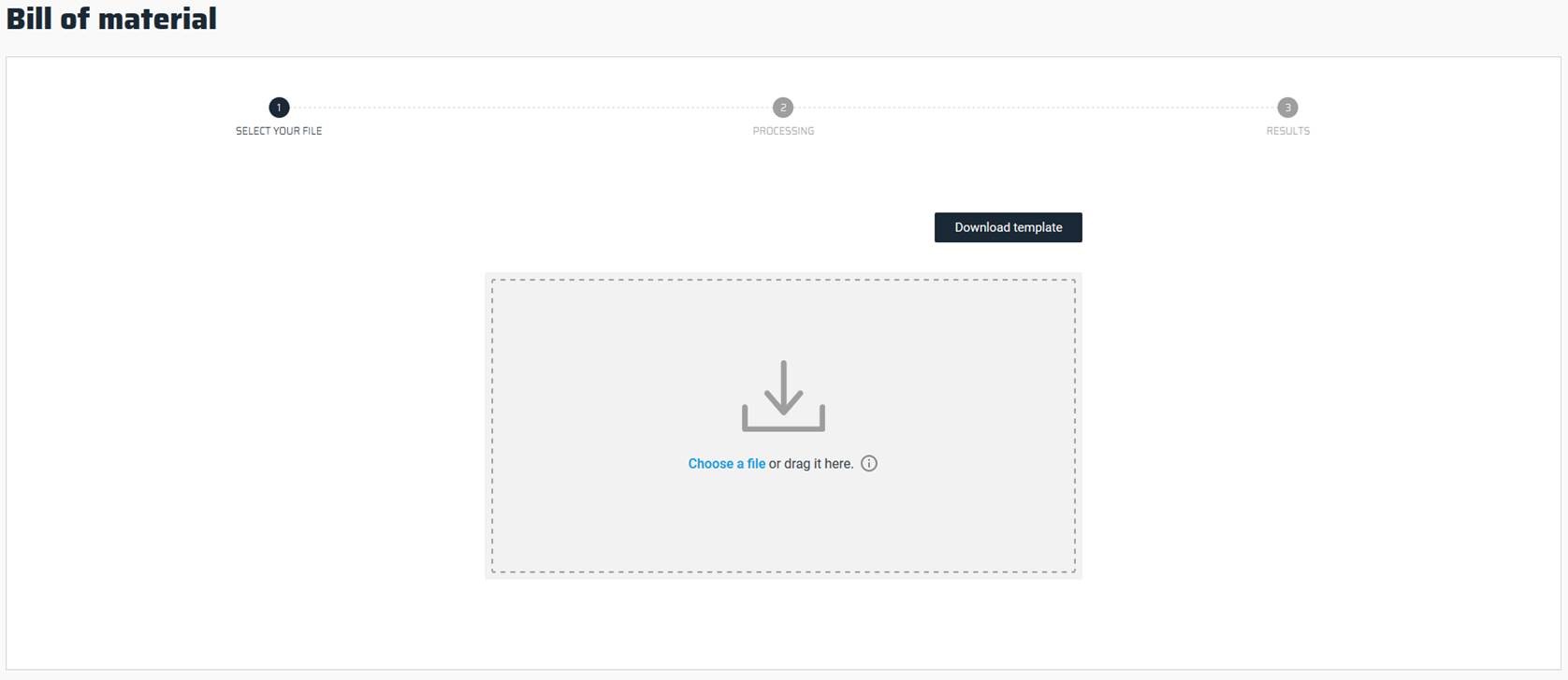This rectangular image, with a width approximately twice its height, features a light gray, almost light blue, border about an inch thick running across the top. In the top-left corner, the bolded black text "Bill of Material" is prominently displayed. A thin gray border frames the image along the left, right, and bottom edges.

Centered in the upper portion of the white background, about two inches from the left, is a small black circle containing a white number "1". Below this circle, the text "SELECT OR FILE" is written in black, all capital letters. A dotted line extends from this circle towards the center of the image.

At the center, a gray circle with a white number "2" inside it denotes the "PROCESSING" step, also in all capital letters. Another dotted line stretches from this circle towards the right side of the image.

Further to the right, about two inches from the edge, a gray circle contains a white number "3" beneath which the text "RESULTS" is written in gray, all capital letters. Between the circles labeled "2" and "3," and situated about two inches down, is a black tab with the text "DOWNLOAD TEMPLATE" in white.

Directly below the number "2", there is a light bluish, light grayish square outlined with darker gray dotted lines. Within this square, a download icon is displayed, and below it, in blue text, "CHOOSE A FILE" is written, followed by the black text "or drag it here." Additionally, a circle with an "i" inside of it is also present in the image.